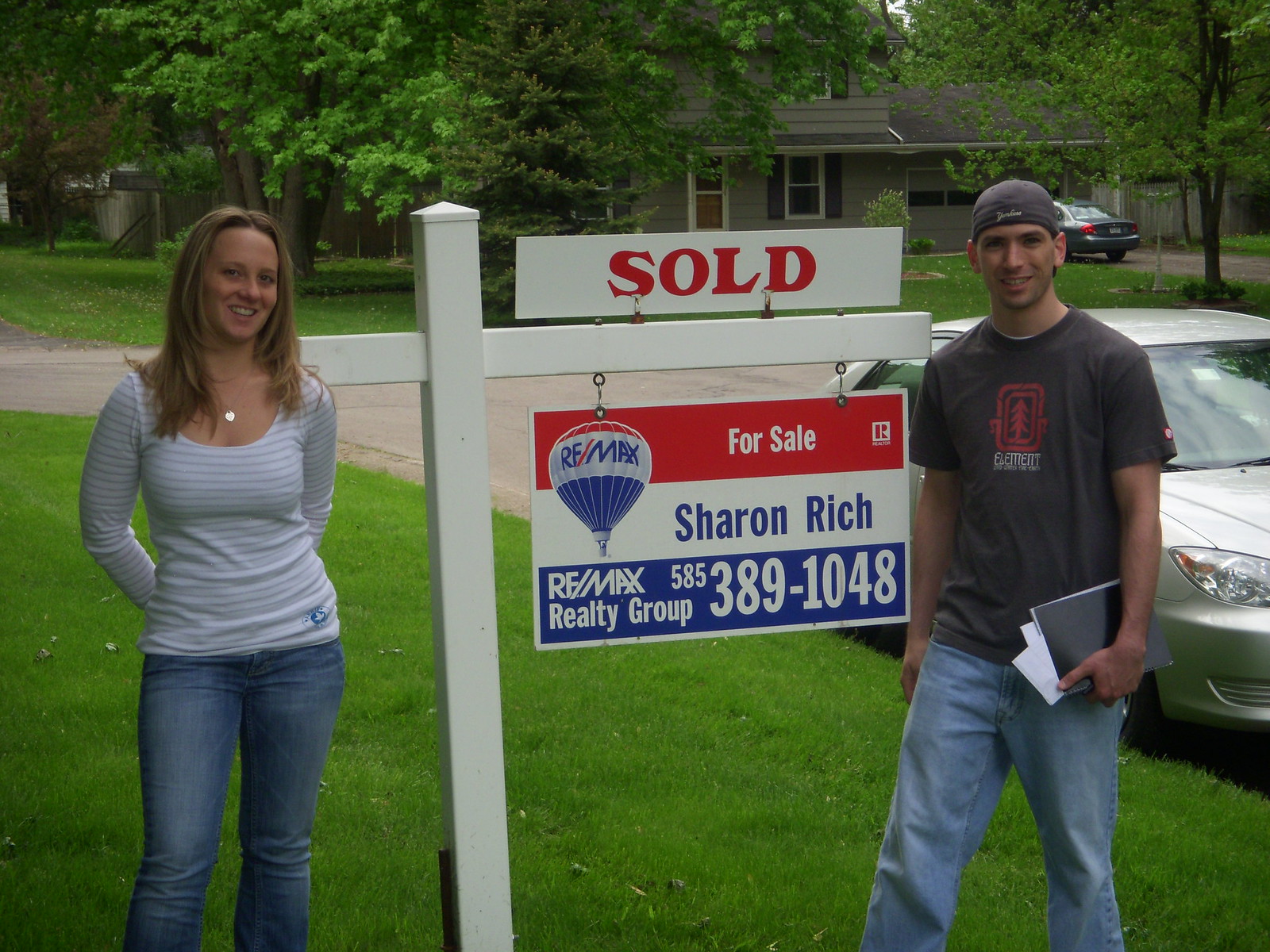In the image, a smiling couple stands in front of a "Sold" sign from RE/MAX Realty Group, likely indicating they have just purchased a house. The scene is set in a yard with vivid green grass and a gray pavement street visible on the right, where their silver car is parked. The RE/MAX sign is prominently displayed with a white pole structure; it has a rectangular white background with bold red "Sold" text, beneath which is a multi-sectioned main sign. The top section is red with "For Sale" in white text, the middle is white with "Sharon Rich" in blue text, and the bottom is navy blue featuring the RE/MAX balloon logo and the contact information "RE/MAX Realty Group 585-389-1048."

The woman, a younger Caucasian with long blonde hair, stands on the left. She is dressed in a horizontally-striped, light-colored top, blue jeans, and has her hands clasped behind her back. The man, standing to the right, is a white male wearing a backwards gray baseball cap, a dark gray short-sleeved shirt, and blue jeans. He holds a black folder with white papers in his left hand. The overall joyful demeanor of the couple suggests their excitement about their new home purchase.